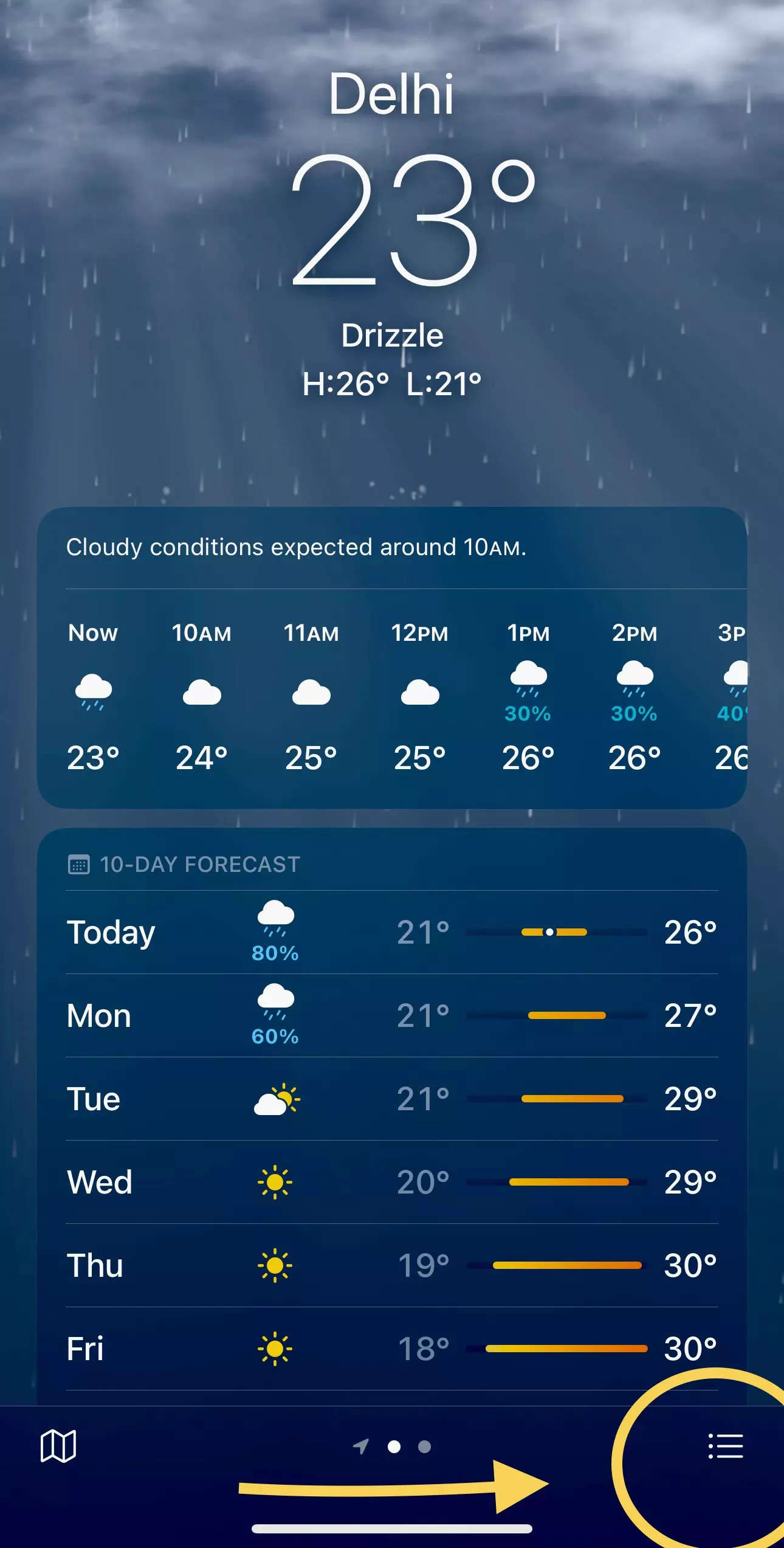**Detailed Caption:**

This image is a screenshot from the iPhone Weather app displaying the weather forecast for Delhi. The current temperature is 23°C, with a drizzle. The forecast for today includes a high of 26°C and a low of 21°C. At 12 PM, the temperature will rise to 25°C, and from 1 PM to 3 PM, it will reach the day's peak at 26°C, accompanied by rain. The app displays an 80% chance of rain today and a 60% chance tomorrow, which is Monday. The forecast for Tuesday predicts partly sunny weather, while Wednesday, Thursday, and Friday are expected to be sunny. The bottom of the screenshot features a yellow arrow pointing towards the menu bar, enclosed by a circle, suggesting this is the section to click for adding or changing the city.